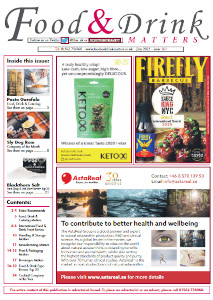**Newsletter Front Page: "Food & Drink Matters"**

The front page of the newsletter titled "Food & Drink Matters" prominently features the title in bold with the ampersand and the word "Matters" highlighted in cranberry red. Below the title, the layout is divided into a long vertical box on the left and three smaller boxes arranged horizontally on the right.

**Left Vertical Box:**

- Header: "Inside This Issue"
- **Image 1:** A vivid photograph of a white bowl filled with a deliciously prepared pasta dish.
- **Image 2:** A cozy scene of someone pouring a beverage from a sleek black bottle into a paper cup, set against a plaid blanket backdrop.
- **Contents List:** The newsletter contents are listed here with article titles in bold black font and page numbers highlighted in red.

**Right Horizontal Boxes:**

1. **Top Box - Keto Advertisement:** A green bag of seaweed chips prominently displayed as a Keto-friendly snack option.
2. **Middle Box - Firefly Barbecue Advertisement:** An enticing ad for Firefly Barbecue featuring a bottle of barbecue sauce with a vibrant label in yellow, blue, and red, alongside a delectable serving of barbecue chicken.
3. **Bottom Box - Astereel Advertisement:** 
   - Header: "Contribute to Better Health and Well-Being"
   - **Images:** Three different pictures of waterways and activities such as outdoor events and a close-up image of an eye, symbolizing holistic health and well-being.

This detailed and visually engaging layout captures the reader's attention, highlighting the key features and advertisements within the newsletter.